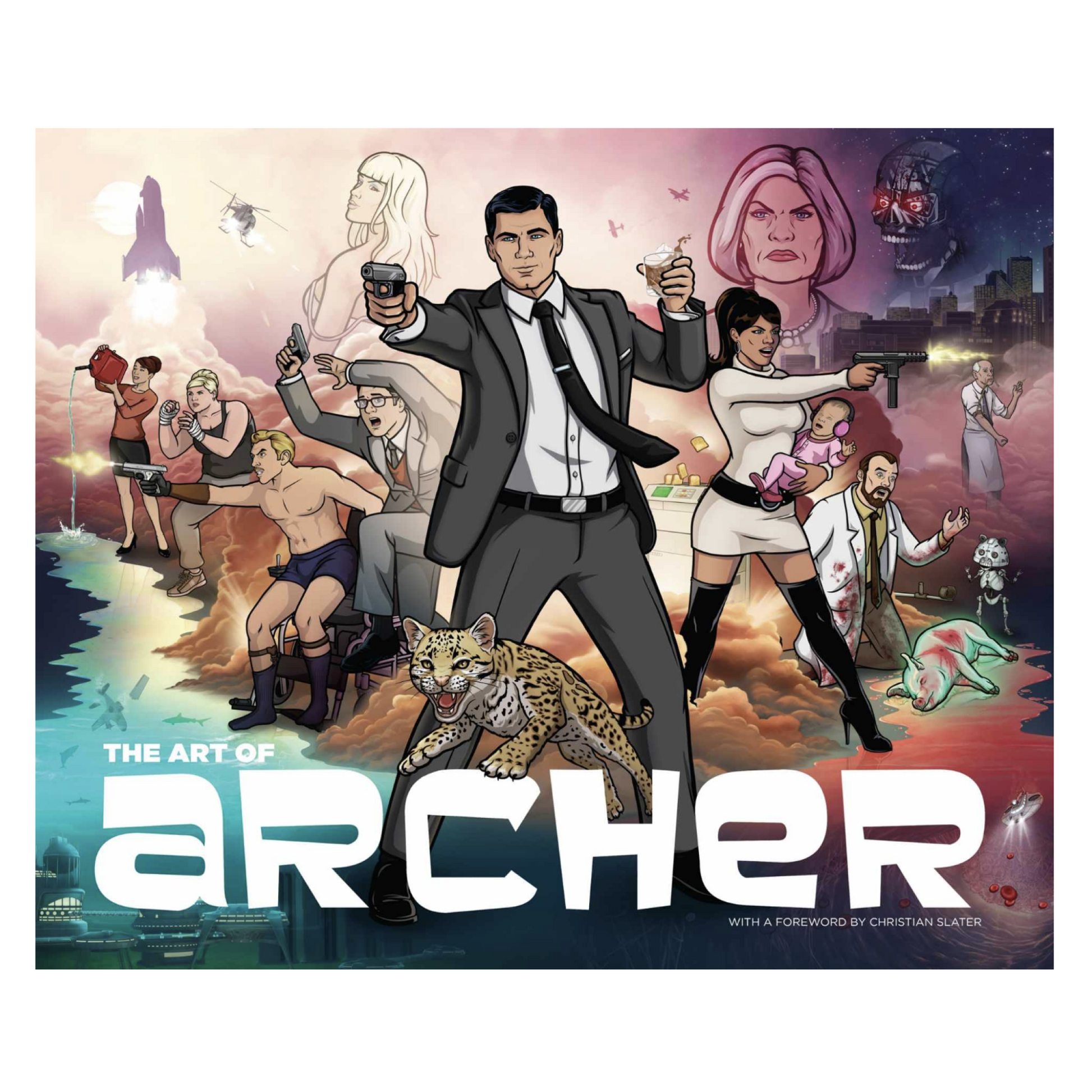This image is a highly detailed and dynamic collage from the TV show *Archer*, seemingly designed as the cover for a book titled *The Art of Archer*, with a foreword by Christian Slater. The title is displayed prominently in large, stylized white font, complemented by the foreword mention in smaller white print. Dominating the foreground is the main character, Archer, dressed in a sharp black suit with a tie, holding a glass of what appears to be whiskey in one hand and pointing a gun straight at the viewer with the other. Beneath him, a small, spotted jungle cat leaps over the book's title.

A rich array of characters and scenes fills the background, adding depth and intrigue. Notably, there is a woman in a short white skirt wielding a gun, a man in swimsuits also armed, and a lady humorously holding both a baby and a firearm. A doctor kneels in front of a dead pig, his lab coat stained with blood. Adding to the chaos, someone is pouring water from a gasoline tank.

The backdrop features a vibrant, pink, white, and purple sky adorned with various animated elements such as airplanes, helicopters, and a rocket ship. A white castle with a purple top and multiple character cameos are embedded within, enriching the scene. The entire composition captures the eclectic and action-packed spirit of *Archer*.